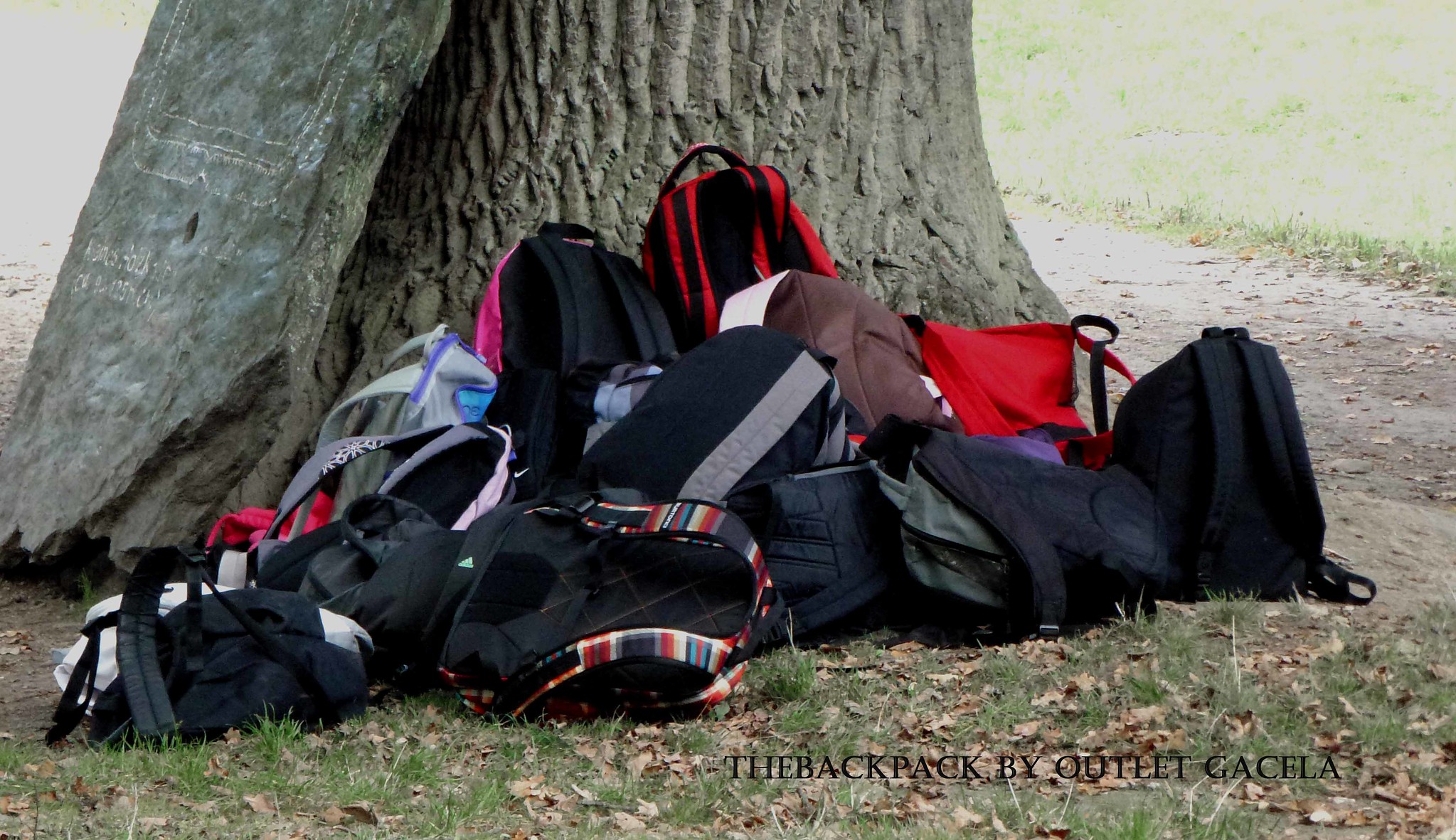This outdoor photograph features a pile of approximately 15 backpacks laid against the base of a large, gray tree trunk. The backpacks display a range of colors including black, red, pink, blue, and plaid-striped designs, some in dual tones such as black and red or black and pink. The scene suggests a high school setting, with the backpacks resting on a grassy area scattered with dead leaves, possibly indicating fall. In the background, there is a mix of dirt, mud, and a lightly washed-out grassy field under bright light. Additional details include a carved stone on the left, a chalk drawing resembling a smartphone on another nearby tree, and a path on the right side of the image. A watermark in the bottom right corner reads, "The Backpack by Outlet Gacela."